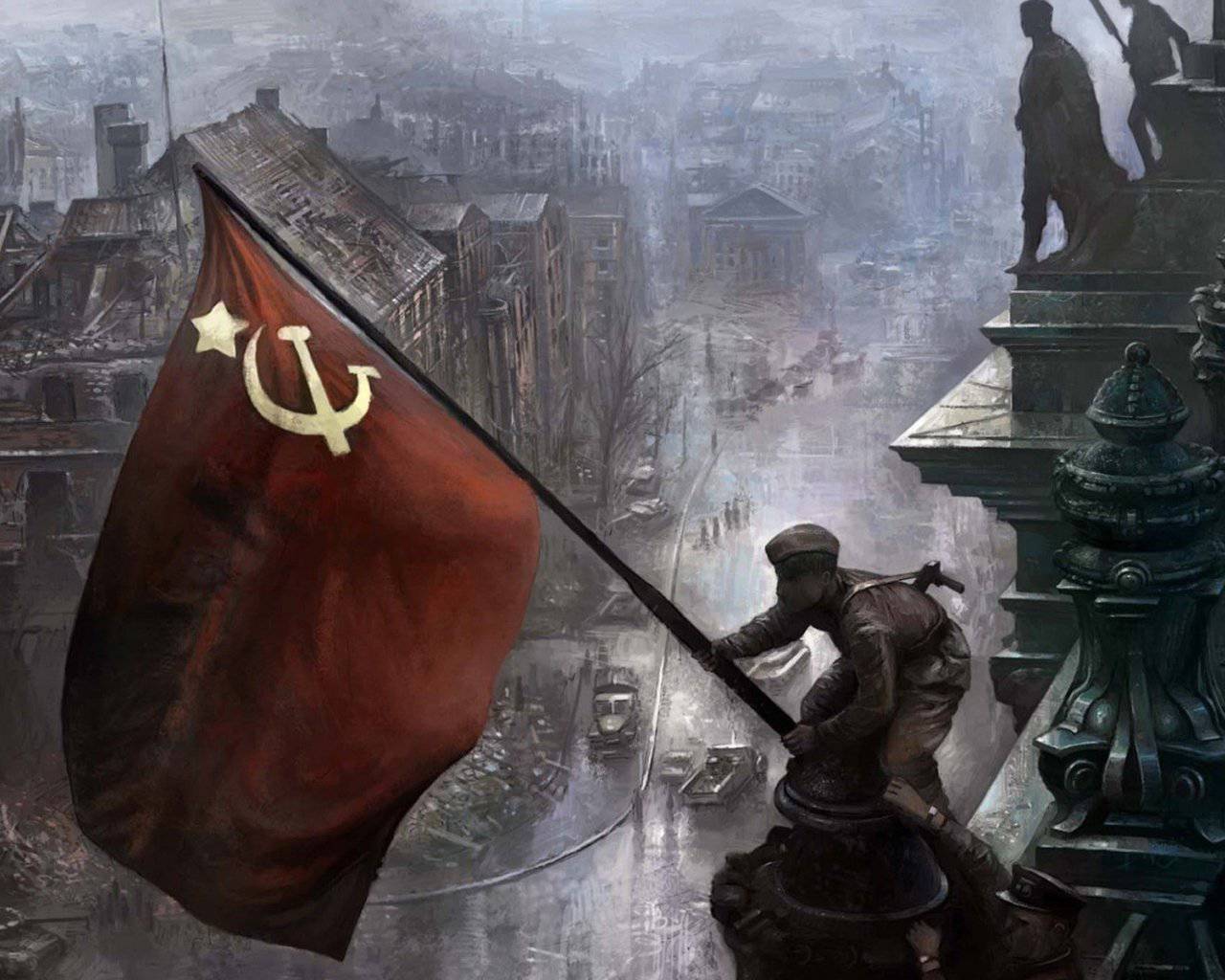The painting depicts a grim, war-torn cityscape from the vantage point atop a building. Dominating the scene is a statue of a Soviet soldier hoisting the Soviet flag, vibrant in red with yellow accents, signifying its historical significance amidst the black and white surroundings. The soldier, clad in an old-school Soviet Union uniform, stands resolutely establishing the flagpole. Below, the city is shrouded in a smoky and dark ambiance. The buildings are largely in ruins, with numerous structures appearing damaged by fire or bombs, and some missing roofs entirely. The scene captures the chaotic aftermath of war, with a winding road where old cars and four tanks are stationary, while a handful of soldiers and a few civilians tread through the desolate street. The wet, shiny ground suggests recent rainfall, enhancing the gloomy and oppressive atmosphere that pervades the city.